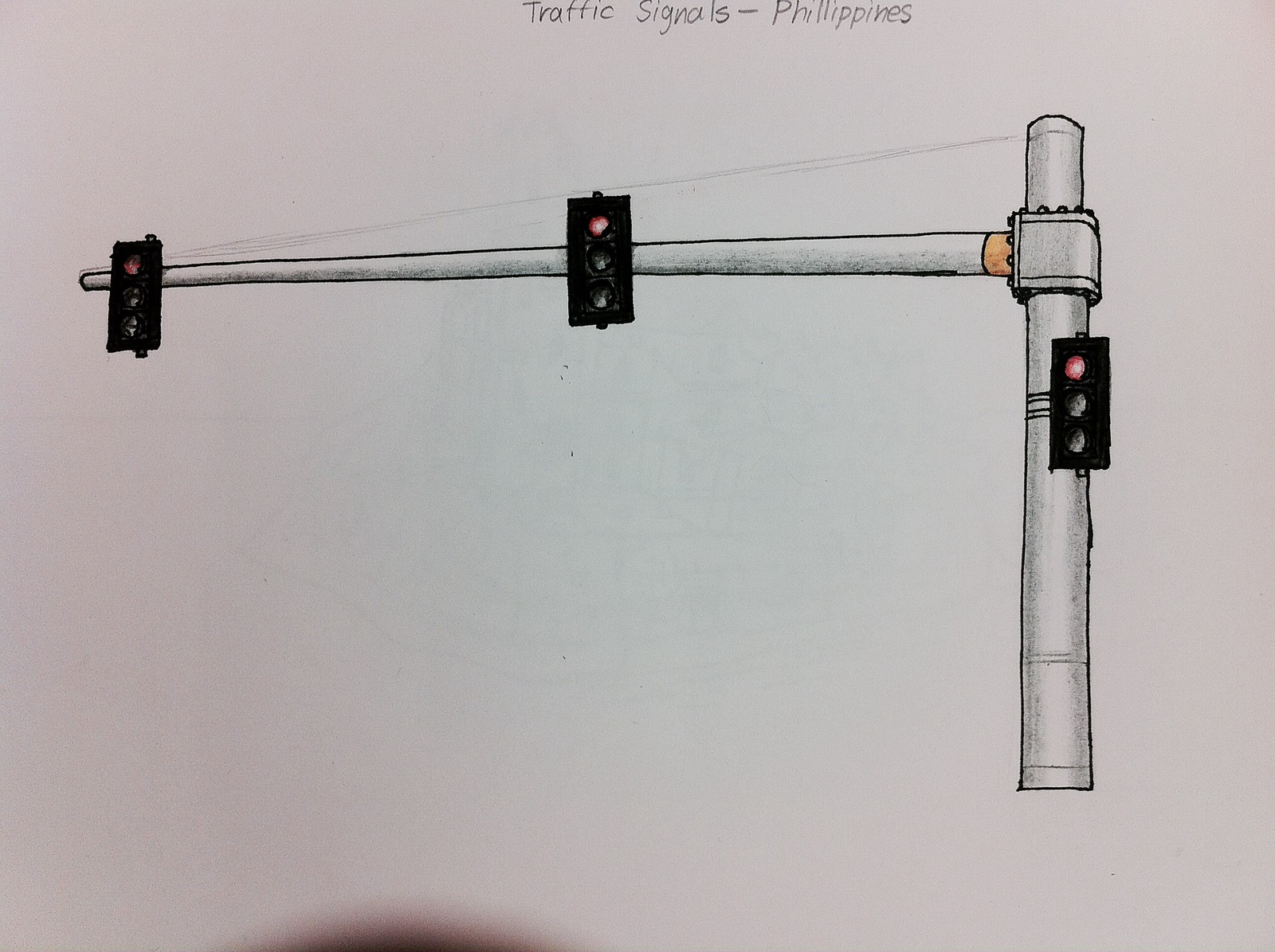This detailed diagram depicts the traffic signal system used in the Philippines. At the top, the title reads "Traffic Signals Philippines." The illustration features three traffic lights mounted on a uniquely designed pole, which is shaped like the number seven or an inverted 'L.' Each traffic light has the conventional arrangement of colors: red at the top, yellow in the middle, and green at the bottom, consistent with the United States' traffic lights. All the lights are currently illuminated in red. The pole supporting these lights is colored gray and includes visible rivets at the joint, emphasizing its robust construction. The entire diagram is presented on a crisp white background, ensuring clear visibility of each component.